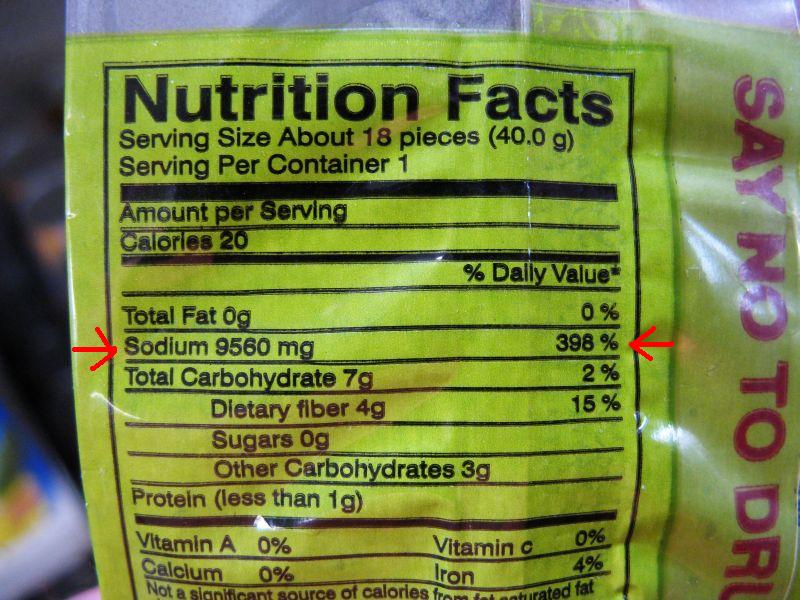The image features a nutrition label with a prominent yellow square that reads "Say No to Drugs." The label emphasizes the high sodium content with arrows pointing directly at the sodium value. The nutritional details are as follows:

- **Serving Size**: Approximately 18 pieces (40 grams)
- **Servings Per Container**: Varies (or more)
- **Amounts Per Serving**:
  - **Calories**: Not explicitly mentioned
  - **Total Fat**: 0 grams (0% Daily Value)
  - **Sodium**: 9560 milligrams (398% Daily Value)
  - **Total Carbohydrates**: 7 grams (2% Daily Value)
    - **Dietary Fiber**: 4 grams (50% Daily Value)
    - **Sugars**: 0 grams
    - **Other Carbohydrates**: 3 grams
  - **Protein**: Less than 1 gram
  - **Vitamin A**: 0%
  - **Vitamin C**: 0%
  - **Calcium**: 0%
  - **Iron**: 4%

Given these values, the label implies that the item is extremely high in sodium, accounting for nearly 400% of the recommended daily intake, which is flagged as particularly concerning.